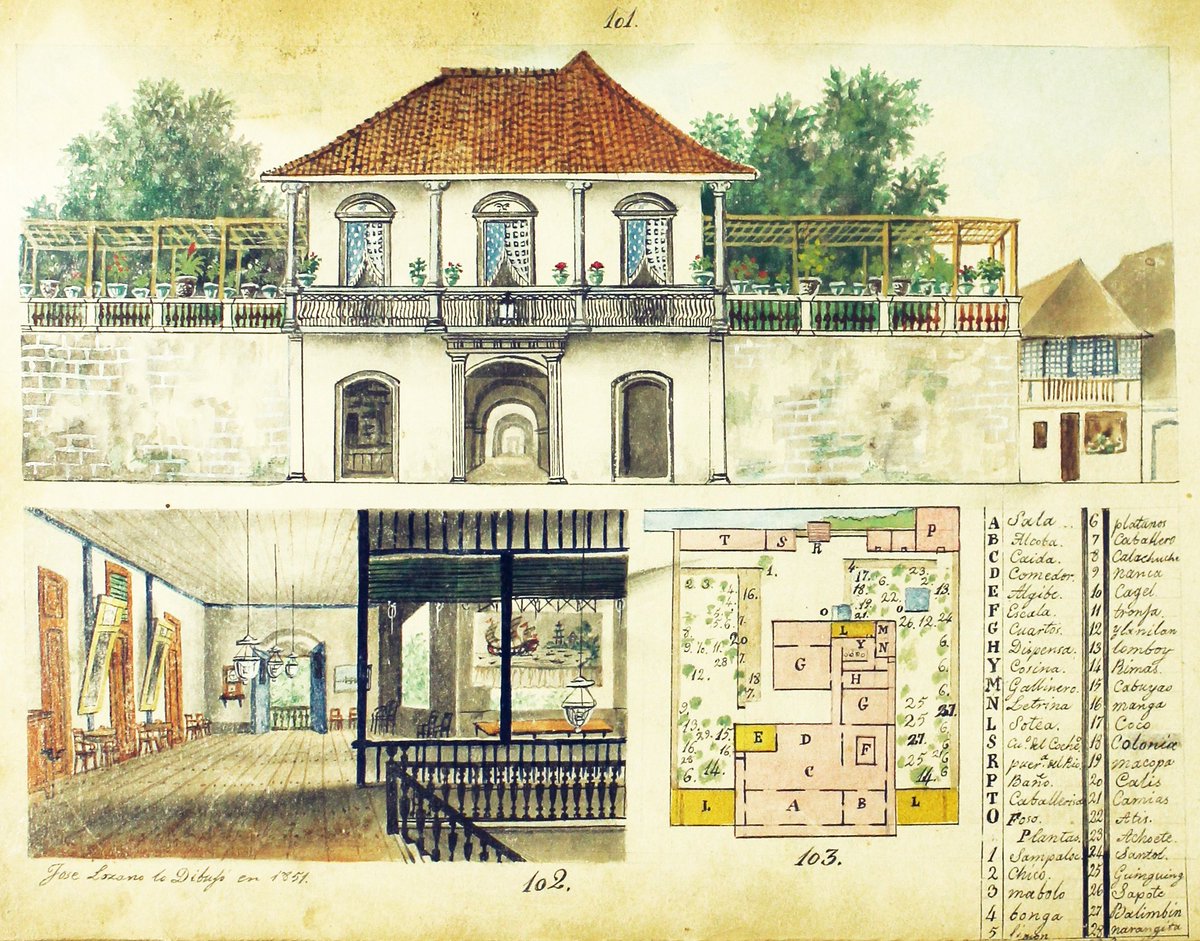The image is an old, colored pencil illustration of a two-story villa-style house, designed to resemble vintage blueprints, possibly dating back to 1851. The paper, now yellowed with age, likely started out white. At the top, there's a detailed depiction of the final design of the house, featuring a brown roof, three walkways at the base, and three windows on the frontal facade. Both sides of the house have awnings and trees, and a white fence runs beneath the house's pillars.

The middle portion of the drawing displays interior views, showcasing black stairs, a wooden-floored room with brown double doors, and another room with blue doors, adorned with paintings and chandeliers. 

The lower part of the page contains the floor plan, with rooms labeled from A to O and numbered from 1 to 28. Each room on the chart corresponds with a detailed description, indicating the function and layout of the spaces. Some rooms are highlighted in pink and green to showcase specific design elements. This illustration serves as an elaborate visual guide of the house, capturing both its exterior design and comprehensive interior layout.